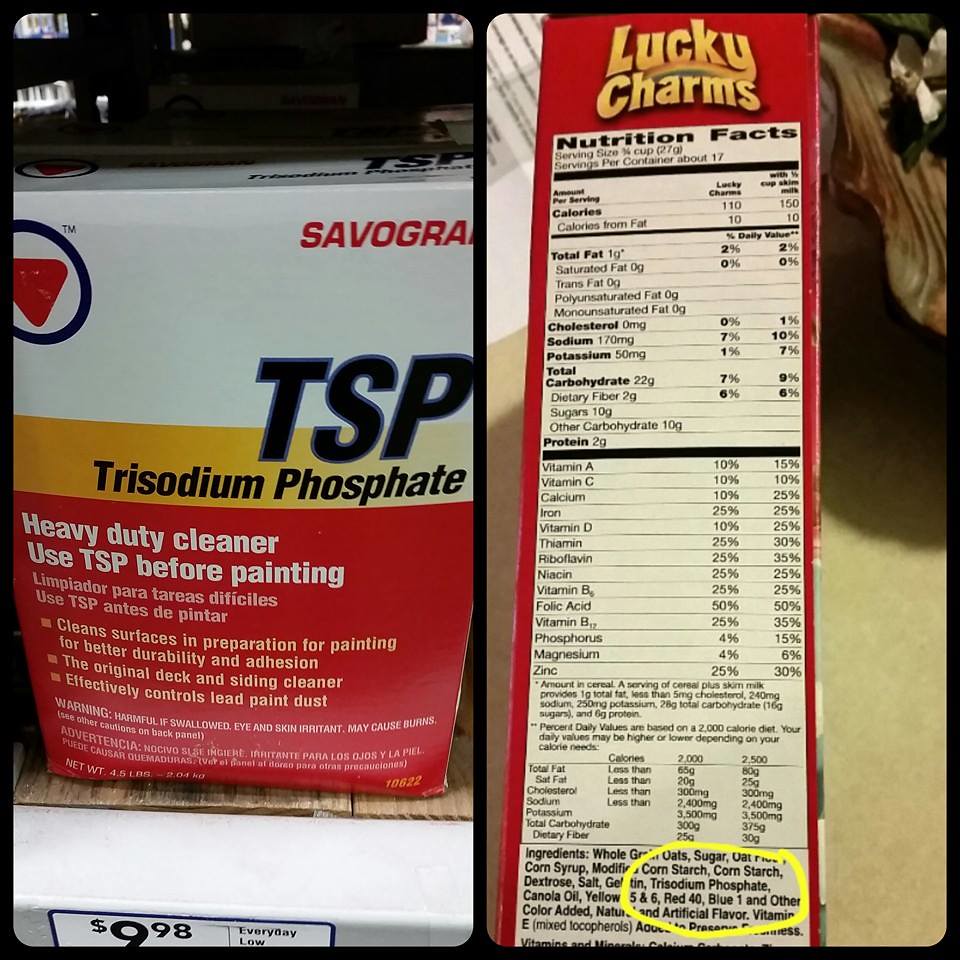The composite image features two juxtaposed photographs. On the left side is a box of TSP, trisodium phosphate, a heavy-duty cleaner commonly used before painting. The box is predominantly white with yellow and red accents, and the label clearly indicates its use for surface preparation in painting. On the right side, the image displays the nutrition facts and ingredients list of a red box of Lucky Charms cereal. The top of the box prominently reads "Lucky Charms," followed by a detailed nutrition chart listing calories, total fat, cholesterol, sodium, potassium, total carbohydrate, protein, sugars, and dietary fiber. Notably, an oval highlight encircles the ingredient trisodium phosphate, the same chemical featured in the cleaner box on the left, drawing a stark comparison between the industrial cleaner and its presence in a food product.